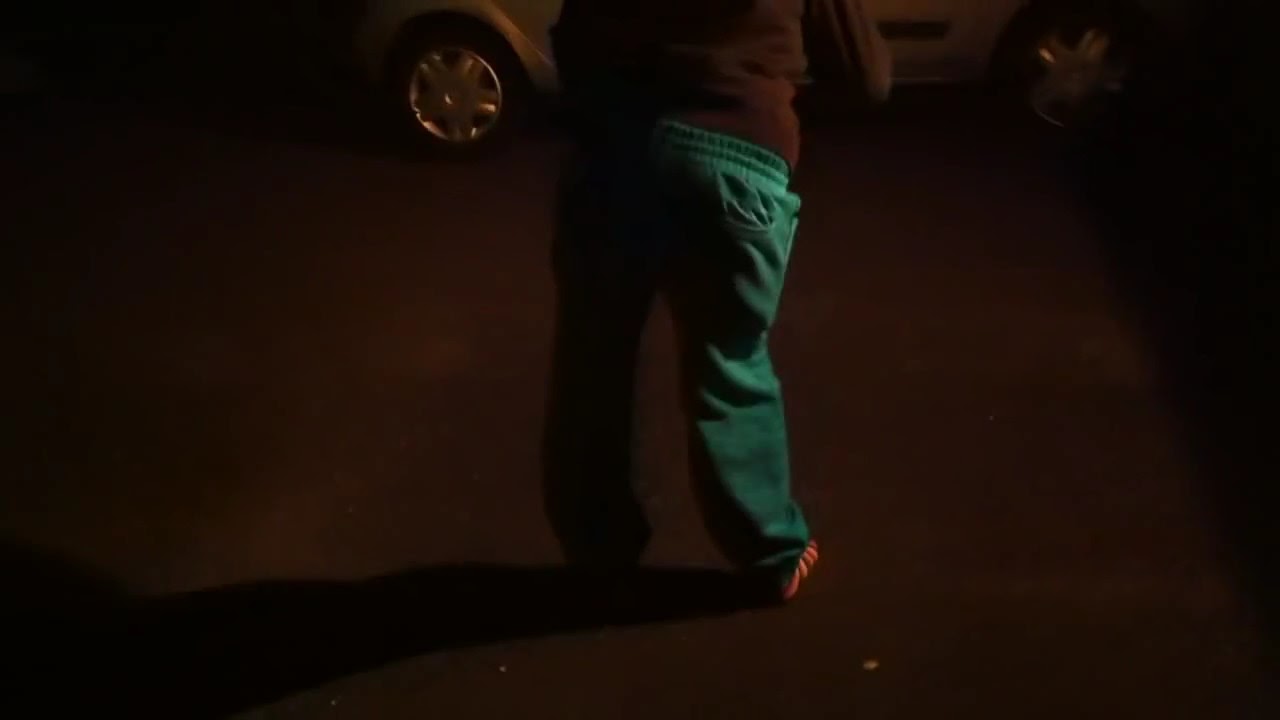The image, taken in the dark at night, depicts a large person standing on a concrete surface, likely a car park. The person's upper body is clad in a brown sweater, with the back of their bent arm visible, ending around the elbow. Below, they wear loose-fitting light to dark green gym trousers that appear skewed, with a pocket on the back. The trousers and an odd shadow on one leg suggest a distorted look due to the lighting. The individual sports striped socks and stands in front of a silver car, part of which—both wheels and part of the body—are visible at the top of the image. A warm white light illuminates the scene from the right, casting the person's shadow to the left.